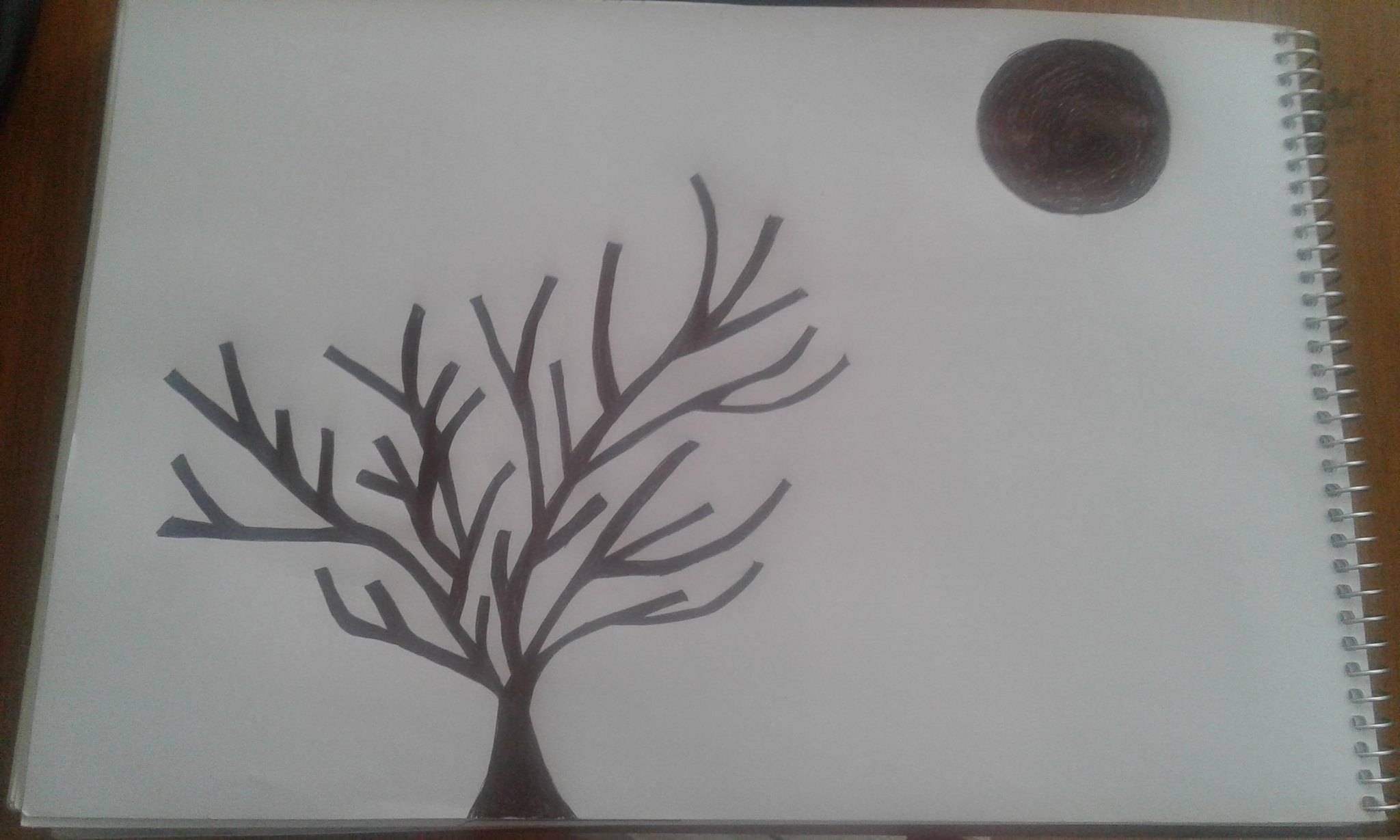This is a detailed sketch rendered on white paper, part of a vertically spiraled sketch pad. The illustration, created using only a dark brown marker, features a barren tree prominently displayed in the center. The tree's intricate structure includes a sturdy trunk that supports several robust branches, which further split into delicate, thinner twigs—all devoid of leaves. In the sky above and to the right of the tree, a large, dark brown circle is depicted, likely representing the moon casting its light down upon the scene. The ground beneath the tree is left empty, focusing attention on the stark, minimalistic beauty of the tree and its lone lunar companion.